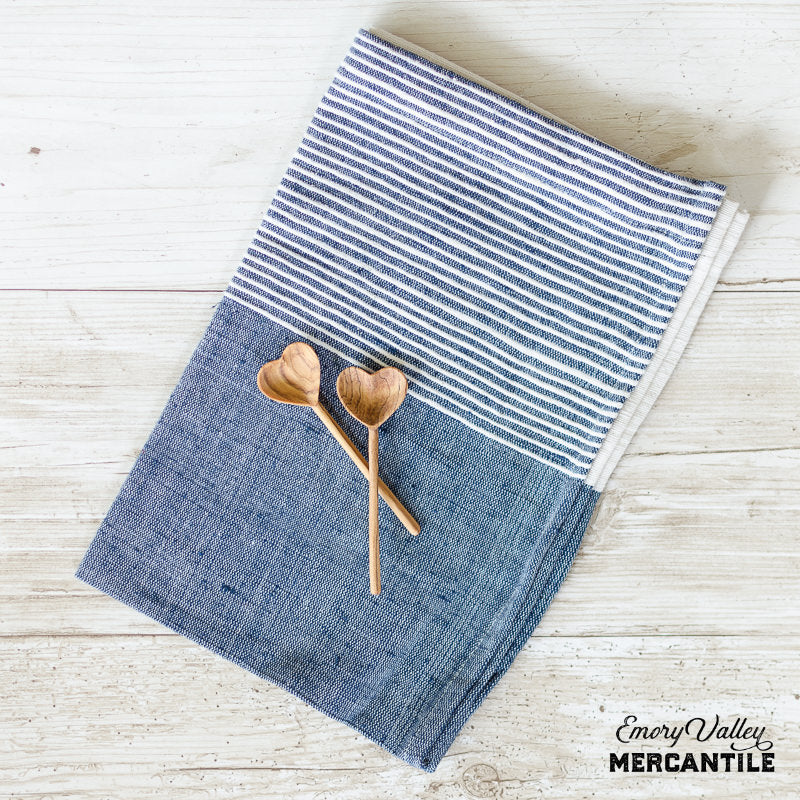This photograph features a folded hand towel set against a white-painted wooden plank background. The towel is divided into two distinct sections: the upper part showcases horizontal blue and white stripes, with approximately thirty thin stripes running horizontally, while the lower portion is a light, denim-like blue fabric. Placed on the blue section of the towel are two intricately carved wooden spoons, with heart-shaped bowls and thin handles, crossing each other. In the lower right-hand corner, scripted in black text, the words "Emery Valley" are visible, with "MERCANTILE" written in thicker black capital letters beneath. This suggests that the items are associated with Emery Valley Mercantile.